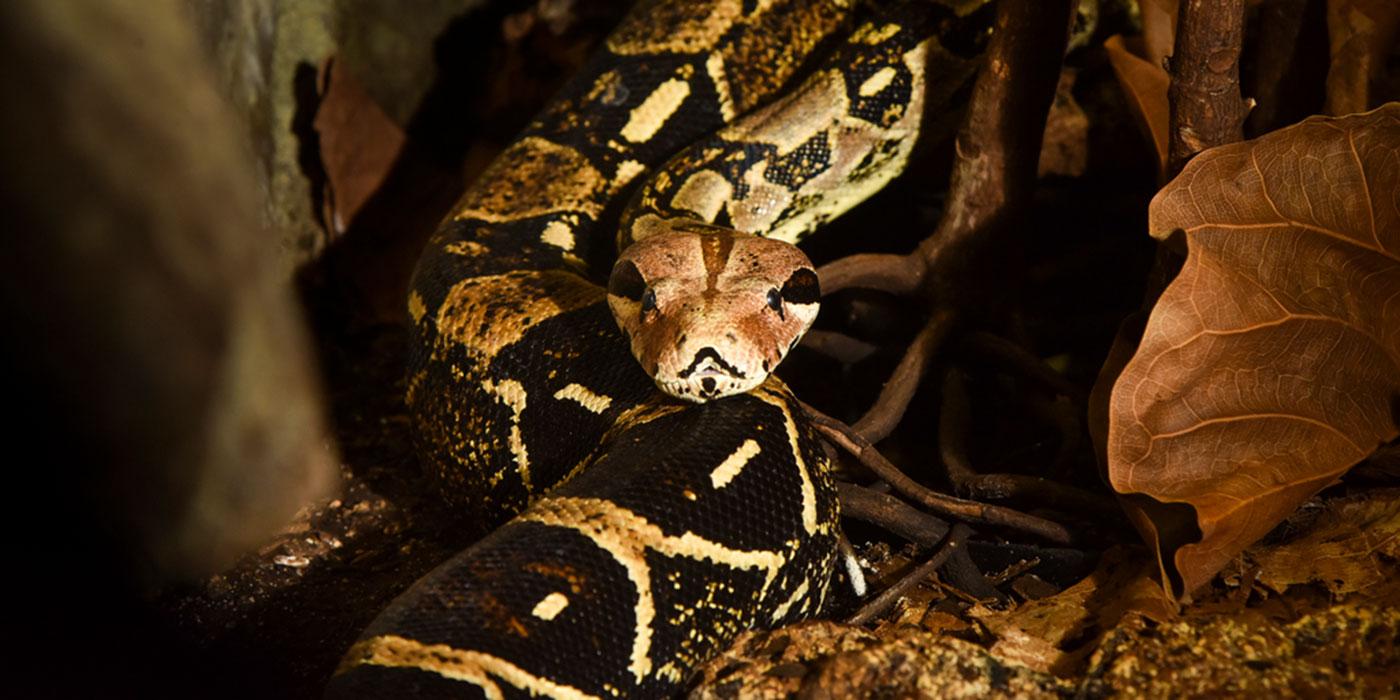In this nocturnal image, a large snake with dark gray or black scales patterned with white zigzag and some tan and brown elements is positioned prominently. Its body stretches away but curls back, bringing its head to the center of the frame, where it stares directly at the camera with suspicious, piercing eyes. The snake rests on a bed of dirt and scattered dried leaves, among which lies a large, brown elephant ear leaf on the right and some green foliage and sticks on the left. The scene, dimly lit with light seemingly from an artificial source to the side, also shows some tree roots in the background, enhancing the forest-like setting. The focused light on the snake creates a stark contrast, accentuating its coiled form and shadow to the left.